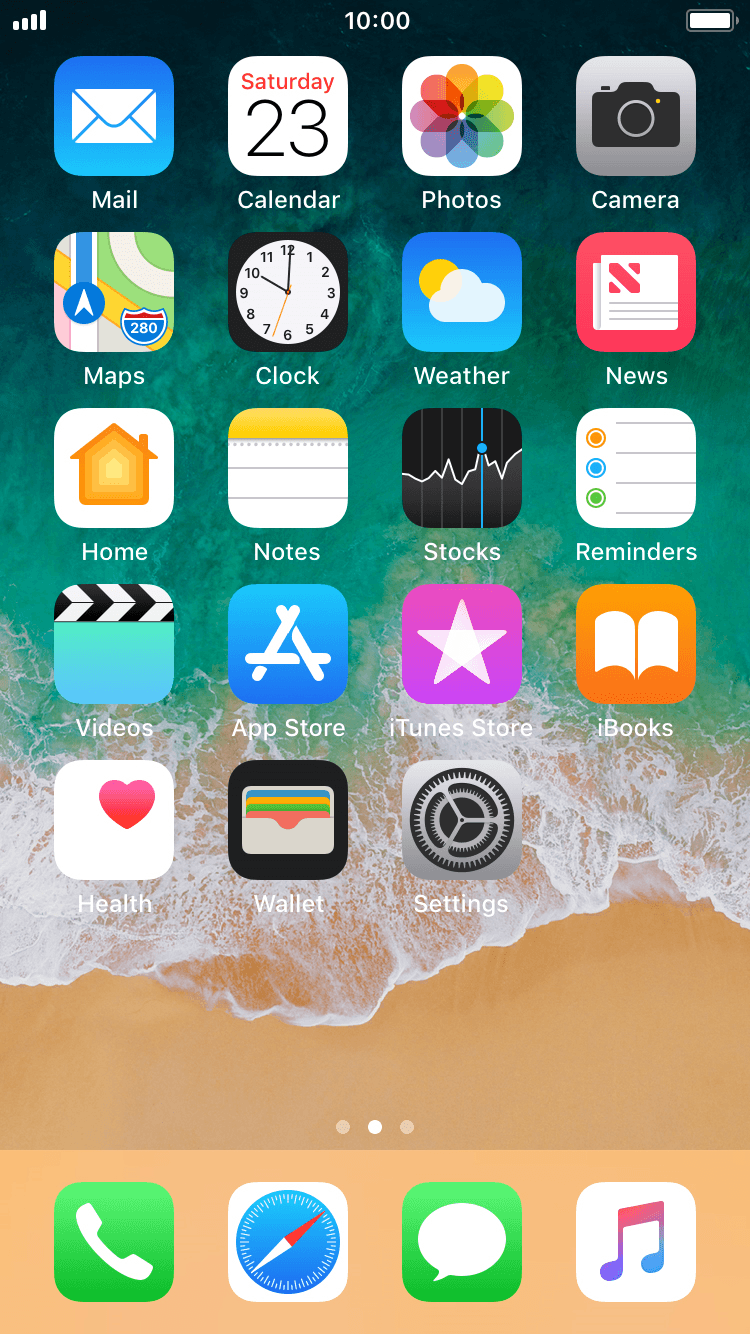The image features an iPhone with a vibrant beach scene as the wallpaper, showcasing a gradient of greenish-blue water transitioning to dark green depths, accentuated by white foam from the waves crashing onto a sandy shore. At the top right corner, the battery life is completely full, indicated by a solid white bar. The time displayed is 10:00, and on the top left corner, the signal bars are completely full, illustrating a strong cellular connection.

The home screen is populated with various app icons meticulously arranged in a grid. Each app icon is distinct, featuring its unique design within a square and labeled in white text below. The visible apps include Mail, Calendar, Photos, Camera, Maps, Clock, Weather, News, Home, Notes, Stocks, Reminders, Videos, App Store, iTunes Store, iBooks, Health, Wallet, and Settings.

At the bottom dock of the screen, four frequently used apps are highlighted: Phone, Safari, Messages, and Apple Music, represented by their respective icons of a phone, compass, speech bubble, and musical note.

The clear detailing of the phone's interface along with the serene beach backdrop creates a striking visual representation of a well-organized and fully functional iPhone screen.